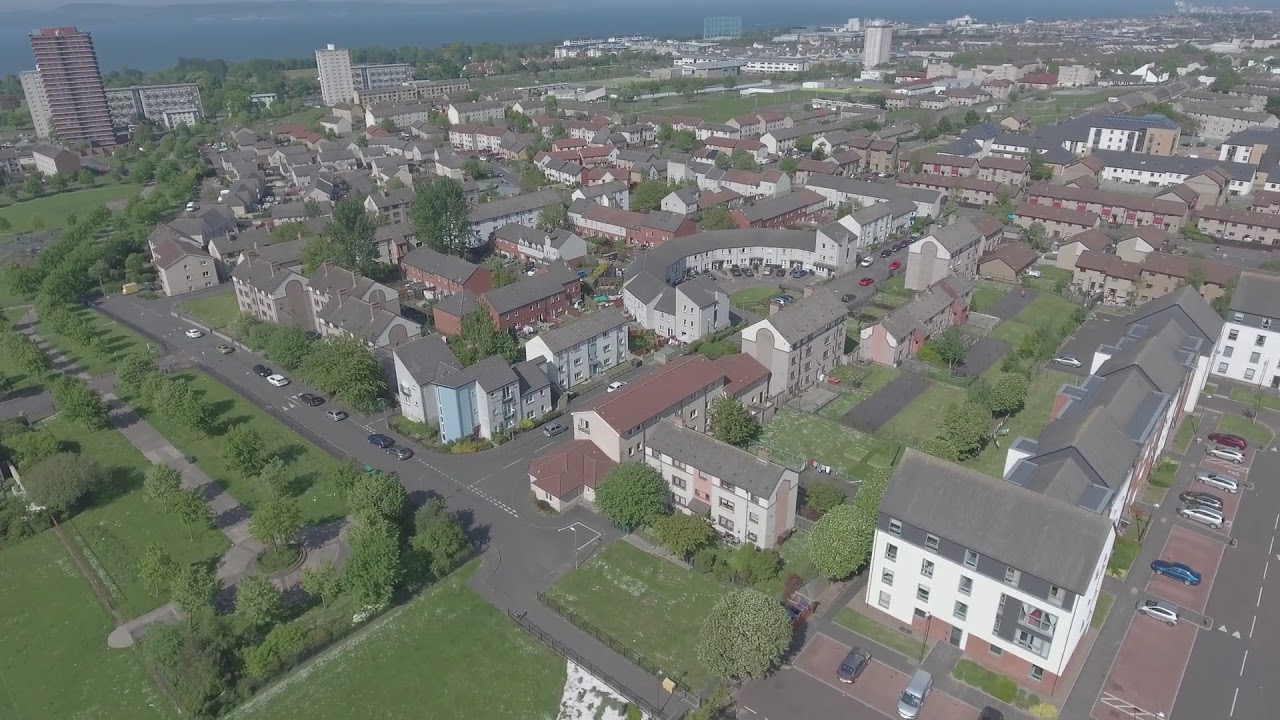This color photograph, taken from an aerial perspective using a drone, captures a detailed view of a small town or village during the day. In the foreground, at the bottom of the image, we can see vibrant greenery comprising bushes, grass, and trees interspersed among roadways and parking areas. The streets meander through the scene, with a prominent main road visible on the lower left side of the image.

Central to this landscape are several multi-story buildings with roofs in shades of gray and maroon, walls predominantly beige and white, suggesting dormitories or apartment complexes. Clusters of similarly styled buildings are arranged in rows, hinting at a residential area with interconnected side streets.

Towards the background, tall high-rise buildings dominate the horizon. Notably, a dark brick condominium tower stands on the top left, approximately 20 stories high, flanked by shorter beige buildings. The top of the image reveals a dark blue sky adorned with scattered clouds, contributing to the outdoor setting's overall serenity. This realistic, photographic representation captures the town's architectural diversity and lush greenery with meticulous detail.